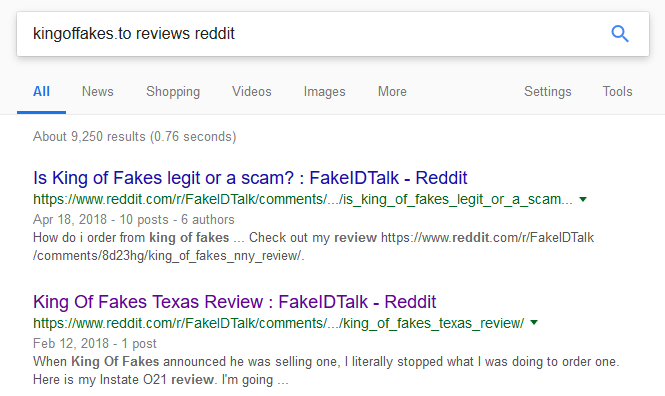Screenshot Description: 

The image is a horizontal screenshot of a Google search results page displaying reviews of the website "kingoffakes.to" on Reddit. At the top, the search bar shows the text "kingoffakes.to reviews on Reddit" has been entered. Below the search bar, the navigation menu includes options for All, News, Shopping, Videos, Images, More, Settings, and Tools.

The search results indicate approximately 9,250 results found in 0.76 seconds. The first result is a Reddit post with the title "Is kingoffakes legit or a scam?" under the "fakeidtalk-reddit" subreddit. The title is highlighted in blue, and the link to the post is in green. Additional information, such as the date of the post (April 18th, 2018), and details about the discussion (10 posts, 6 authors), is presented in gray text. The content snippet reads: "How do I order from kingoffakes? Check out my review," followed by the same link.

The second result has already been visited, as indicated by its purple title. This post is titled "Kingoffakes Texas review" and is also found in the "fakeidtalk-reddit" subreddit. The link is similarly green and includes the URL "https://www.reddit.com" repeated twice.

The image captures all these details, providing a comprehensive snapshot of the search results for "kingoffakes.to reviews" on Reddit.